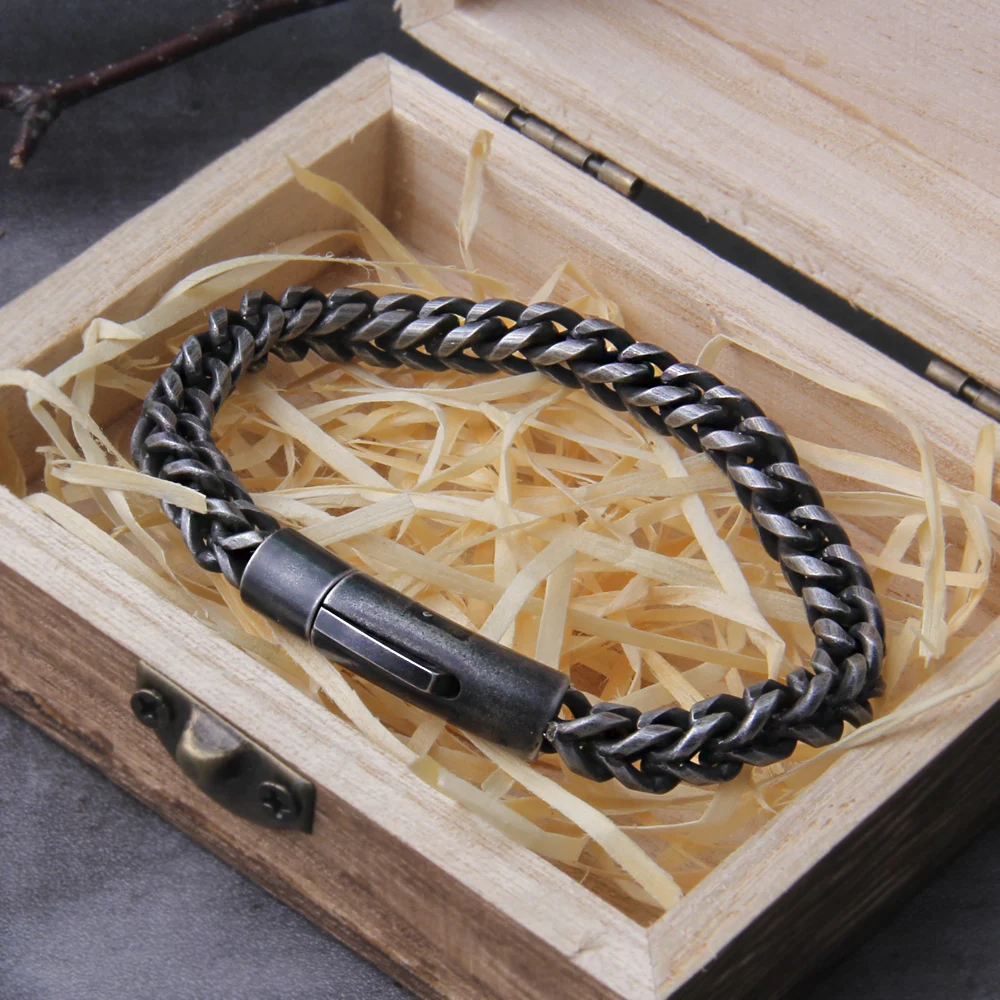The image features a meticulously crafted metallic bracelet nestled inside a small, unfinished wooden box. The bracelet itself is designed with interlocking metal rings, reminiscent of chainmail, suggesting a high level of craftsmanship. The metal is polished, giving it a refined appearance, and includes a cylindrical centerpiece with a lock mechanism and a large button for opening. The bracelet is presented on a bed of light beige straw, adding a touch of rustic elegance.

The wooden box is unpainted, emphasizing its handmade quality. It has a straightforward construction with thin metal hinges and a small metal latch secured by two screws on the front. Adjacent to the box, there is a stick, and the entire composition rests on a gray surface with a similar gray background, enhancing the focus on the bracelet and its packaging.